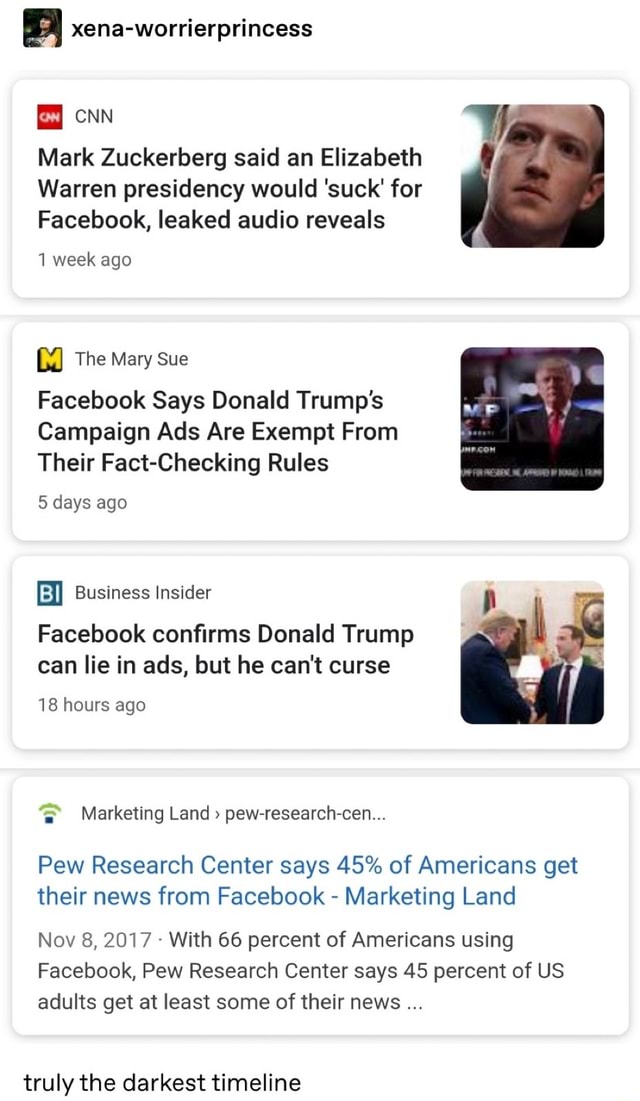The image features various text fragments and graphical elements presented in a collage-like format. At the top, there's text that reads "Xena: Warrior Princess." Below, another section contains a red square with rounded corners displaying text that says, "CNN: Mark Zuckerberg stated that an Elizabeth Warren presidency would suck; Facebook leaked audio reveals," dated one week ago. Adjacent to this, there is an image of Mark Zuckerberg and another text block labeled "The Mary Sue," discussing Facebook exemptions from fact-checking rules credited to John Charles Campinas, dated five days ago.

Additionally, there's a blurred background image featuring Donald Trump, overlaid with text from Business Insider referring to a Facebook conference and humorously censored language, timestamped 18 hours ago. Another square with rounded corners near the bottom left reads, "Pew Research Center: 45% of Americans get their news from Facebook," accompanied by a marketing statistic from 2017 stating that 66% of Americans use Facebook. At the bottom, a text suggests, "45% of your sales get at least some of their news," concluding with the phrase, "Truly the darkest timeline."

The overall collage combines these elements to present a chaotic yet insightful commentary on Facebook’s influence, media coverage, and political implications.